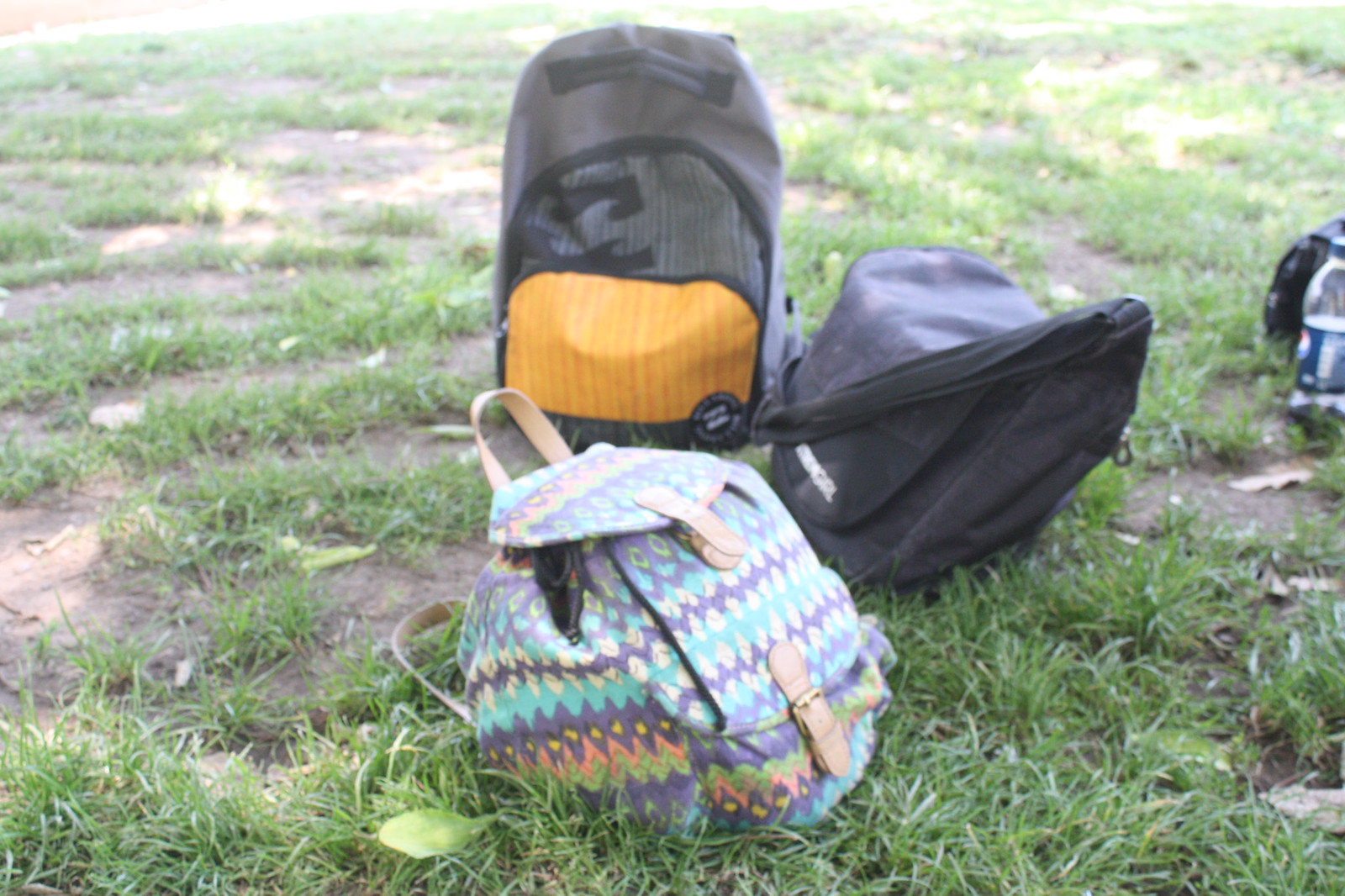This photograph, taken on a sunny day in what seems to be a park, shows a patchy expanse of grass dotted with dirt and leaves, indicating a less maintained area. In the center of the image are three backpacks, casually placed. The foremost backpack is colorful with pink and blue stripes and a zigzag pattern, featuring distinctive leather toggles and a pair of sunglasses peeking out. Slightly behind, to the left, is a black messenger bag with an unreadable white inscription. To its right is a standard backpack with a yellow outer pocket and grey body. Notably, at the very right edge of the picture, an empty, upright Pepsi bottle is partially visible. The scene suggests a recently abandoned picnic or outdoor gathering.